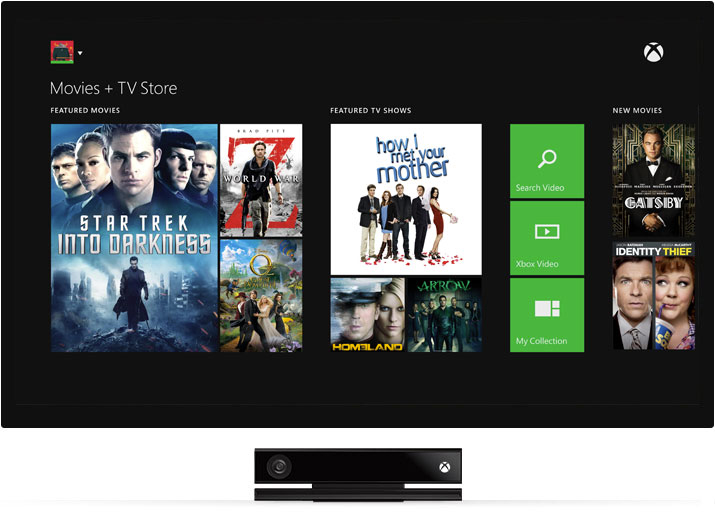This is a screenshot of the Xbox interface, highlighting various sections of the Movies and TV Store. In the top left corner, there's a profile photo that's too small to identify. Directly below this is the "Movies + TV Store" heading, followed by the "Featured Movies" section, showcasing "Star Trek Into Darkness," "World War Z," and "Oz." Among these, "Star Trek Into Darkness" is prominently displayed with the largest title and corresponding movie poster.

To the right is the "Featured TV Shows" section, which includes "How I Met Your Mother," "Homeland," and "Arrow," with "How I Met Your Mother" being the most prominent. Further to the right are options to navigate through the content with "Search Video," "Xbox Video," and "My Collection," each presented within a green square.

To the right of these options is the "New Movies" section, featuring "Gatsby" and "Identity Thief," both with equally sized movie posters. Above this section, in the top right corner, is the Xbox logo. At the very bottom of the image, the Xbox console itself is visible. The interface has a black background with white text, except for the text on the movie posters, which varies depending on the title.